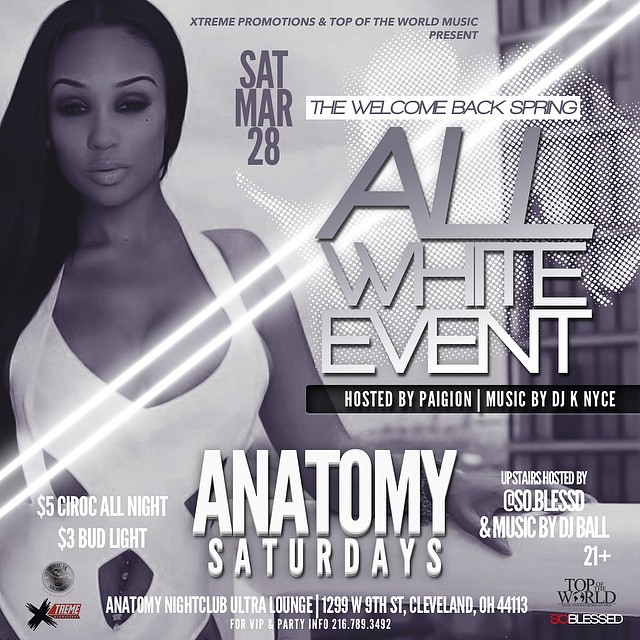The image is an advertisement for a nightclub event titled "The Welcome Back Spring All White Event," hosted by Pagan with music by DJ K Nice. The promotional poster is primarily in black, white, and gray with accents of red. At the top center, it reads "Extreme Promotions and Top of the World Music Present," with a section detailing the event date "Saturday, March 28th" in dark gray font against a white background. Hosted upstairs by At So Blessed, with music by DJ Ball, the event is 21+ and features specials like Ciroc all night and $3 Bud Light.

An African-American woman, possibly in a white one-piece swimsuit that reveals a significant portion of her chest, occupies the left side of the image. She has long, straight black hair that extends past her shoulders and is looking directly at the camera. The event details are densely packed on the right side, stating the venue as Anatomy Nightclub Ultra Lounge, located at 1299 W 9th Street, Cleveland, OH 44113. For VIP and party info, the number 216-789-3492 is provided. The background is predominantly gray, possibly showcasing a building partially obscured by the text. The bottom left and right of the image feature multiple logos, including "Extreme" with a circle, "Top of the World," and "So Blessed," with "So" in red and "Blessed" in white.